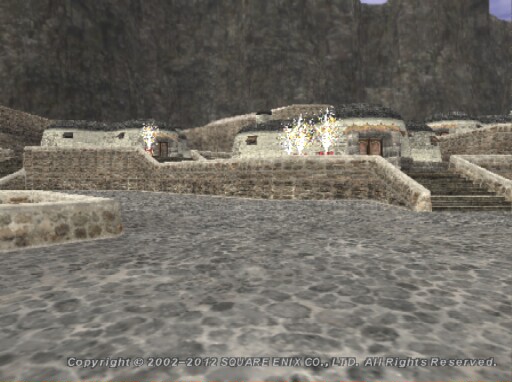This image appears to depict a scene with potential ruins, presenting a blend of elements that might suggest it is a deliberately stylized piece rather than an AI-generated picture. The artistry is somewhat cartoonish in nature. 

The background prominently features a sheer, precipitous cliff that extends from the bottom edge of the image but is cut off at the top, creating a dramatic backdrop. In the foreground, the ground is covered with cobblestone-like stones, adding texture and realism to the setting.

Dominating the middle ground of the image is a central structure that appears to be in ruins, though it is relatively well-preserved. The structure consists of short walls and a small staircase leading up to it. Spread around the central ruins are several smaller buildings or homes, each with discernible doors, evoking a settlement style reminiscent of Tatooine from Star Wars with their humble, utilitarian design.

The image features a text overlay at the bottom that reads, "Copyright 2002-2012 Square Enix Co. Ltd. All Rights Reserved," indicating the possible artistic origins and rights holder of the visual content.